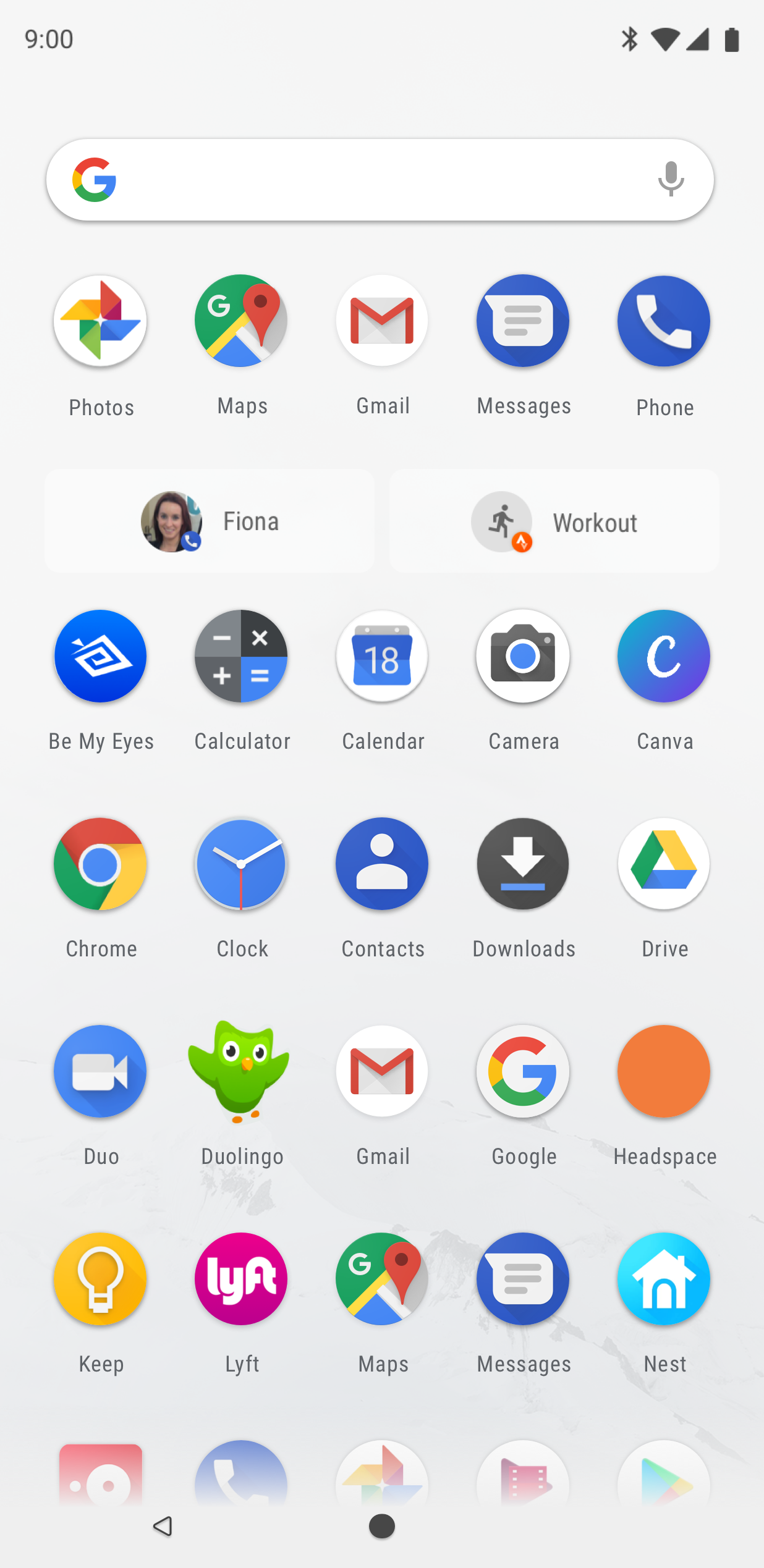The image depicts a cell phone screen displaying the home screen with several visible icons and a Google search bar. At the top of the screen, the time is shown as 9:00, accompanied by standard icons indicating battery life, signal strength, and other common phone statuses.

Beneath the status bar is the Google search bar, featuring the iconic 'G' in red, yellow, green, and blue, and a microphone icon on the right end for voice search functionality. 

The first visible row of app icons includes a photo app, Google Maps, Gmail, Messages, and a phone app. Following these is a section featuring a profile picture of a woman labeled "Fiona" next to an icon of a person running, marked "Workout," which also indicates one new notification.

Below this section, there is an array of app icons: 
- "Be My Eyes"
- Calculator
- Calendar
- Camera
- Canva

Proceeding to the next row, the icons include:
- Google Chrome
- Clock
- Contacts
- Downloads
- Google Drive

Continuing downward, the following apps are lined up:
- Duo
- Duolingo
- Gmail
- Google
- Headspace

Moving further, the icons displayed are:
- Google Keep
- Lyft
- Google Maps
- Messenger
- An icon marked "Next"

The final visible row of app icons is partially cut off, revealing only the top parts of the icons without any descriptive labels.